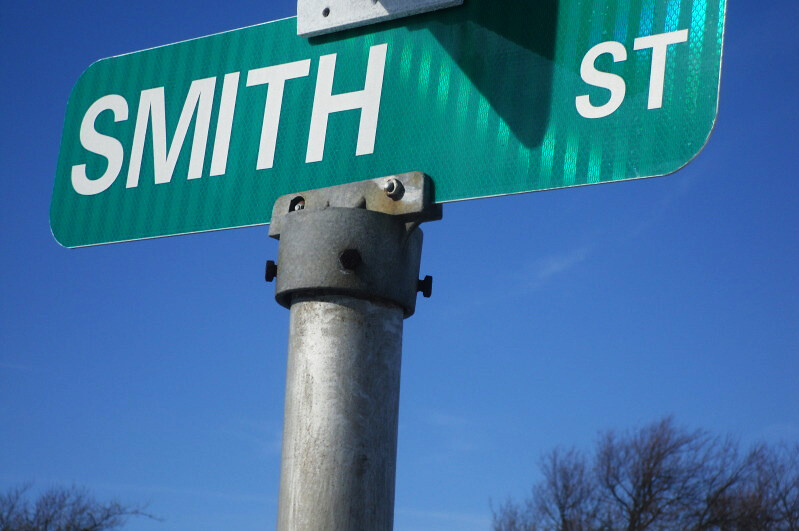The image captures a vibrant street scene, with the centerpiece being a rectangular green street sign displaying the name "Smith Street." Photographed from a low angle, the sign is set against a clear, azure sky that fills the background. Adding a touch of nature, tree branches extend into the sky, partially framing the sign. The street sign is affixed to a sturdy, gray metal pole, noticeable for its robust construction. The top of the pole features a circular bracket secured by visible screws, which support a horizontal bar that stabilizes the sign. A shorter metal piece, also gray, extends horizontally above the "Smith Street" sign, further anchoring it to the pole.